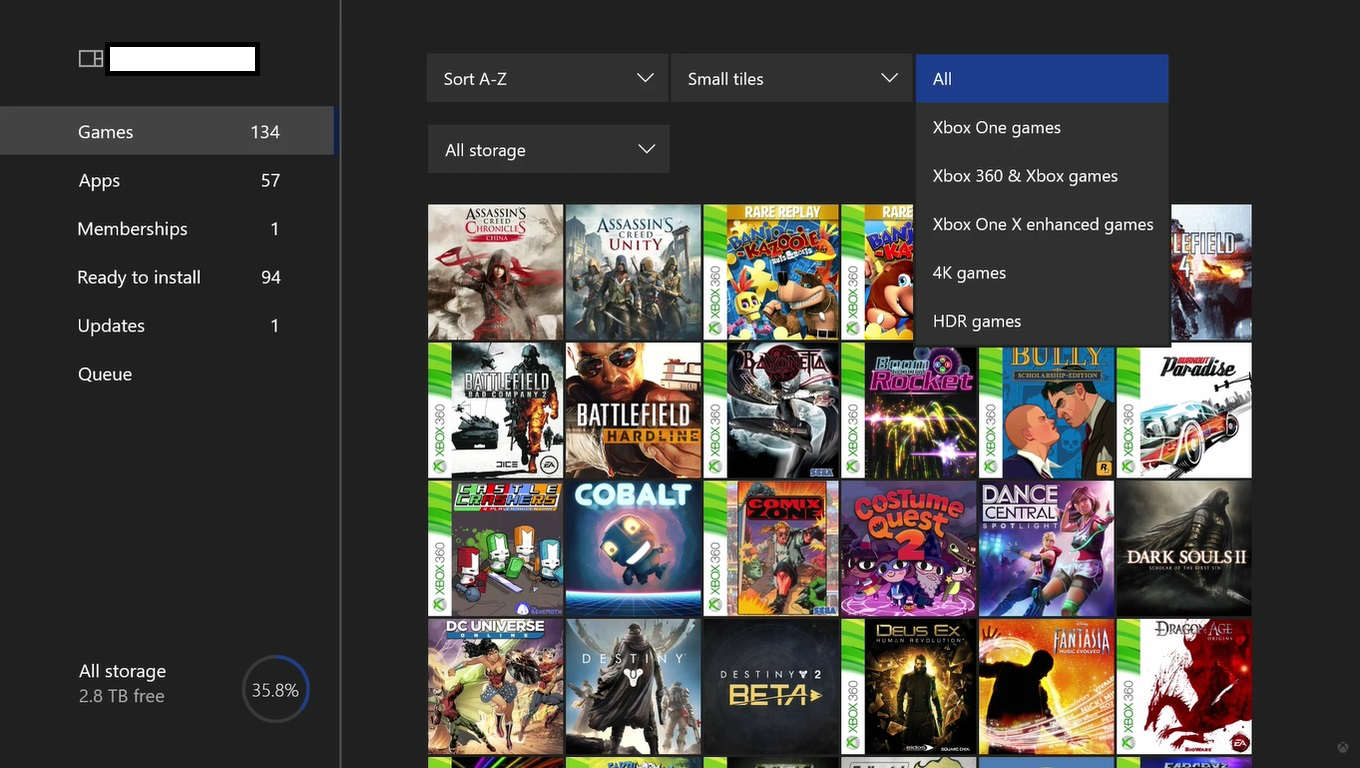The image appears to be a screenshot of a gaming platform interface. In the upper left corner, there is a rectangular search box for finding specific content. Immediately below this search box is a list of clickable categories, which include: "Games," "Apps," "Memberships," "Ready to Install," "Updates," and "QA." Each category has a number beside it indicating the quantity of items in that section. At the bottom left corner of the screen, there is a storage status display indicating "2.8 TB free," accompanied by a circular graphic showing a usage percentage. 

On the right side of the screen, there is additional clickable information, including an arrow icon. This section also showcases a variety of game covers, each with a vibrant and colorful design. The covers display the titles of the games, and there are multiple options available to the viewer. At the top of this section, it appears that the filter "All" has been selected, allowing the user to browse different types of games.